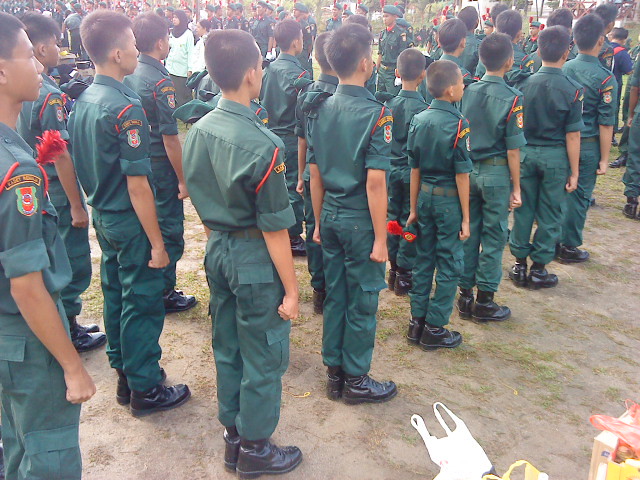This digital photograph captures an orderly line formation of young boys and adolescents who appear to be of Asian descent, possibly Vietnamese. They are dressed in kelly green paramilitary-style uniforms, complete with black boots and uniforms that feature orange accents and a badge on the sleeve. All the boys have dark, very short hair. The ground they stand on is barren, with only a few patches of grass visible, indicating a rugged outdoor environment. In the foreground, particularly at the bottom right of the image, lie a white bag, an orange bag, a yellow bag, and a cardboard box. The young boys are positioned in the front of the formation, with taller, older boys standing behind them. The day appears to be bright, and in the backdrop, there are other individuals in similar green uniforms, as well as civilians, including a woman in a white shirt and black headscarf, which adds depth to the scene.